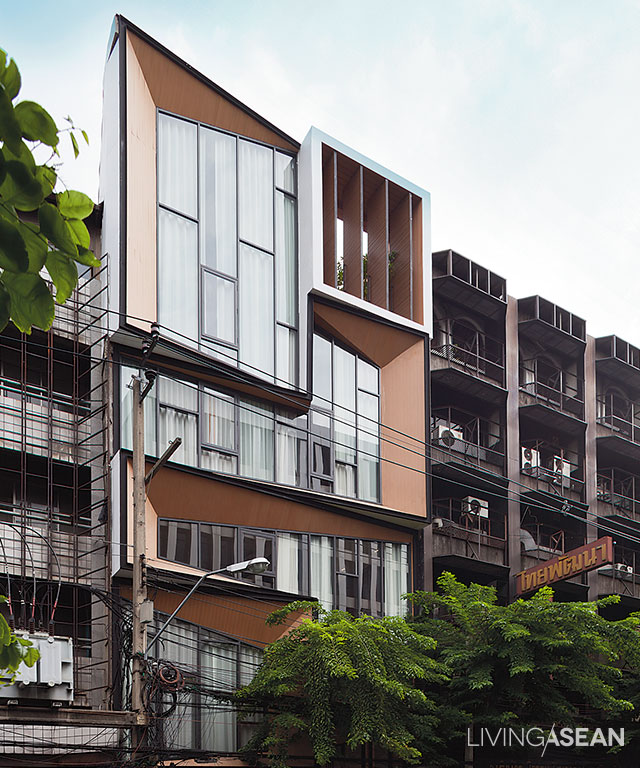This photograph, taken outdoors, captures a street scene in a foreign country, likely to be in a warm or tropical environment due to the presence of lush green trees and palm-like plants. Three distinct buildings dominate the image: 

On the far left, a three-story structure made of gray concrete is evident, surrounded by metal scaffolding, suggesting ongoing construction or refurbishment. It lacks windows and looks rather industrial.

In the middle, the tallest building showcases a modern design. It features a glass front accentuated with brown borders, large floor-to-ceiling windows, and balconies. This building has notable brown accents around the windows and a somewhat louvered appearance at the top. It's framed by more green foliage, likely indicating spring or summer.

The building on the right, slightly traditional and seemingly run down, has visible air conditioners on its balconies, hinting at a hot climate. This structure includes aspects like fans and large windows, contributing to the image's overall warm, lived-in feel.

A street pole with a lamp, which appears outdated compared to the modern middle building, and several power lines crisscrossing in front of the buildings add to the urban setting. The sky above is a mix of blue and cloudy, enhancing the photograph's natural atmosphere. A watermark at the bottom-right corner reads "Living A.S.E.A.N."

The entire scene is enclosed within a vertically oriented rectangular frame.